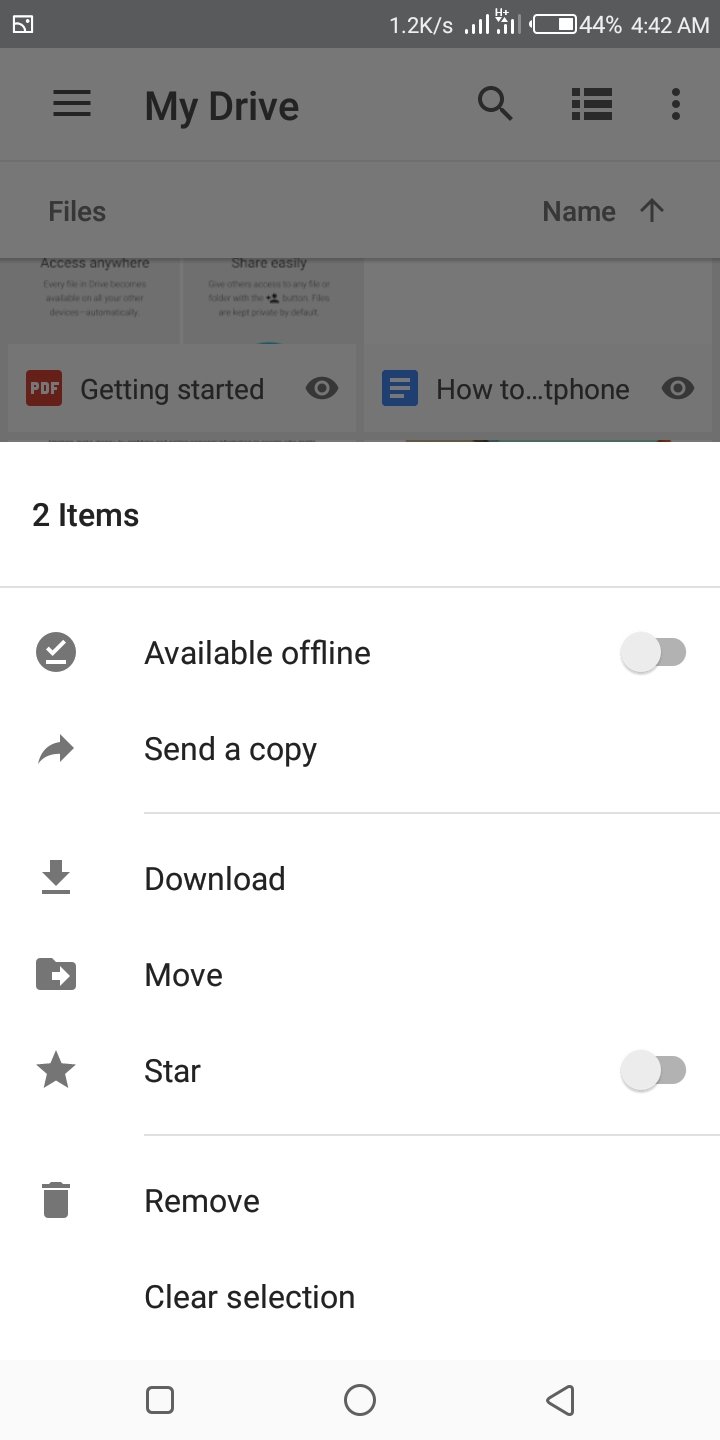### Descriptive Caption

**Screenshot of a Mobile Device Interface**

The upper section of the screenshot displays a gray status bar with notable details: the topmost line is a darker shade of gray, indicating system status. It shows a strong internet connection, 44% battery life, and the current time, 4:42 a.m., suggesting that the phone should be charged soon. 

Within this gray status bar, several icons and text elements are visible:
- A hamburger menu on the left.
- The text "My Drive" in a large black font.
- A magnifying glass icon for search functions.
- Another hamburger menu icon with bullet points.
- Three vertically aligned dots for additional options.

Below the status bar, the main content section is titled "Files." This section lists several files, although their full names are partially obscured. The recognizable ones include:
- A PDF titled "Getting Started"
- A document labeled "How To"
- A Word document signified by the partially visible name "t-phone" in blue text.

At the bottom of the file list, it indicates that there are "2 items" available. Options for these items include:
- "Available offline" (currently turned off)
- "Send a copy"
- Icons for "Download," "Move," and "Start" (all aligned to the left and currently turned off)

Further down, there are options to "Remove" (illustrated with a trash can icon) and "Clear Selection." 

Finally, the standard navigation buttons of the phone are located at the very bottom of the screenshot.